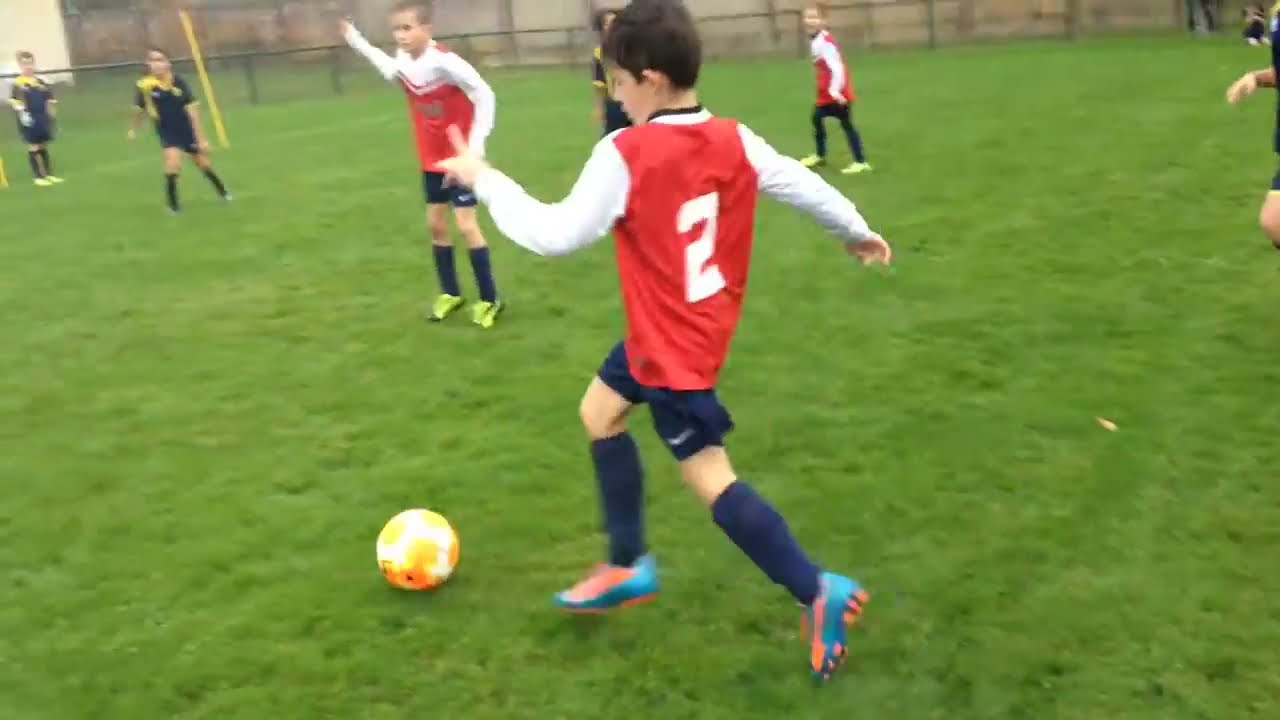The photograph captures an elementary school soccer game set on a vibrant green field. Central to the image is a young boy, likely around 10 years old, poised to kick a gold soccer ball with yellow and orange markings. He is donned in a red jersey with white sleeves and the number two adorning his back, accompanied by navy blue shorts, matching navy blue socks, and striking turquoise cleats with salmon-colored accents and orange studs. The boy's red team, also in Nike-sponsored uniforms, is visible with several teammates scattered across the field. In opposition, players wearing black jerseys with yellow collars, black shorts, and black socks can be seen. Bordering the field is a metal fence, extending from the upper left to the upper right background. The scene includes around seven or eight players, with clear indications of the intense, youthful energy typical of a children's soccer match.